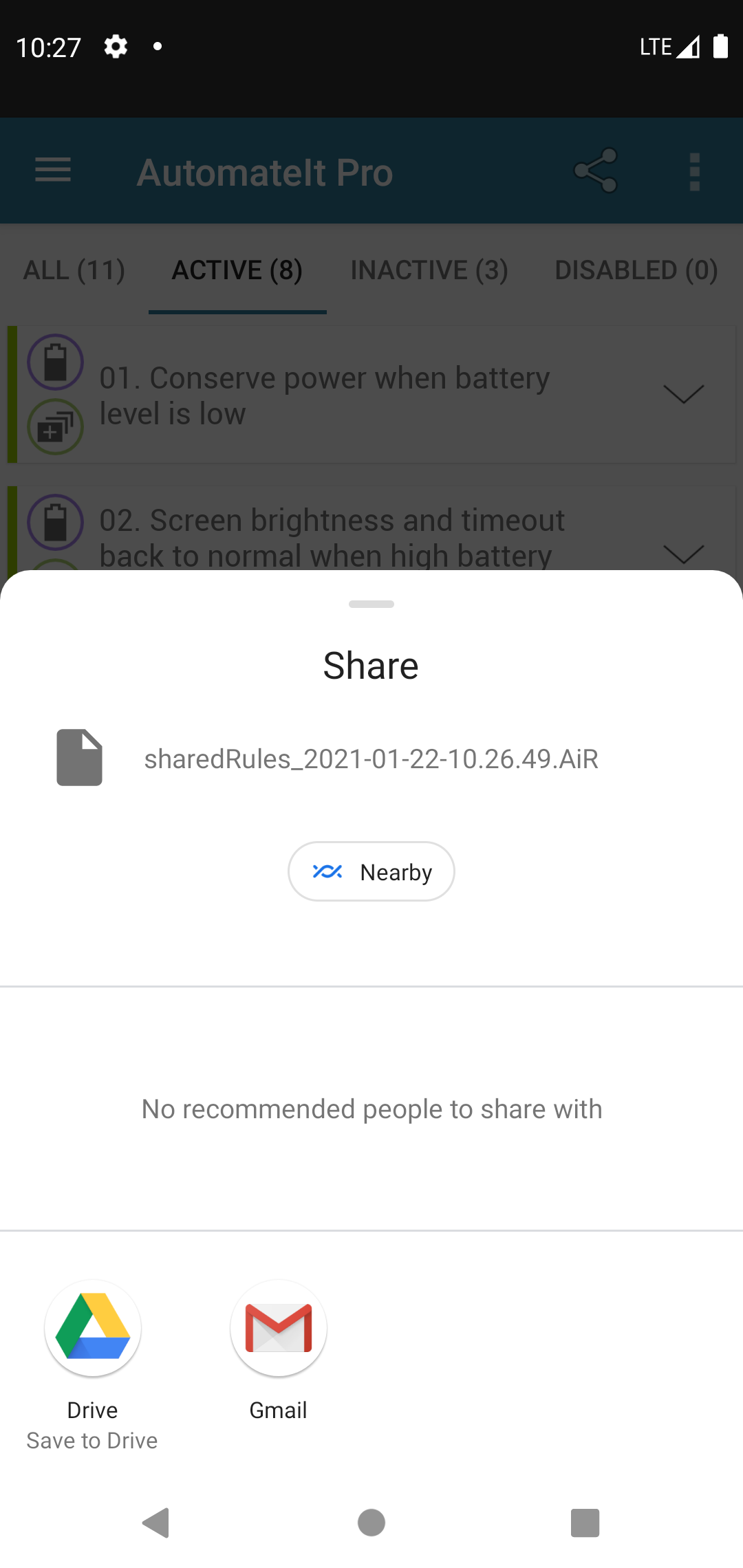The image is a screenshot from the "Automate It Pro" app on a smartphone. It features a pop-up notification in the center that prompts the user to share a file named "shared_rules_2021-01-22-10.26.49.AIR". Below this file name is a button labeled "Nearby". In the background, the main interface of the "Automate It Pro" app is partially visible, organized in a table format with different rows and category tabs.

The visible portion of the app displays two rules:
1. "Conserve power when battery level is low".
2. "Screen brightness and timeout back to normal when high battery".

At the top of the interface, there are multiple category tabs which include:
- "All" with 11 rows.
- "A" with 8 rows.
- "Inactive" with 3 rows.
- "Disabled" with 0 rows.

The tab currently selected is "Active", comprising 8 rows, but only the two aforementioned rows can be seen due to the pop-up overlay.

Additionally, the top bar of the smartphone screen displays the current time as 10:27 AM on the left. On the right, there are several icons indicating system status: a gear icon, a battery icon, a Wi-Fi indicator, and an LTE indicator.